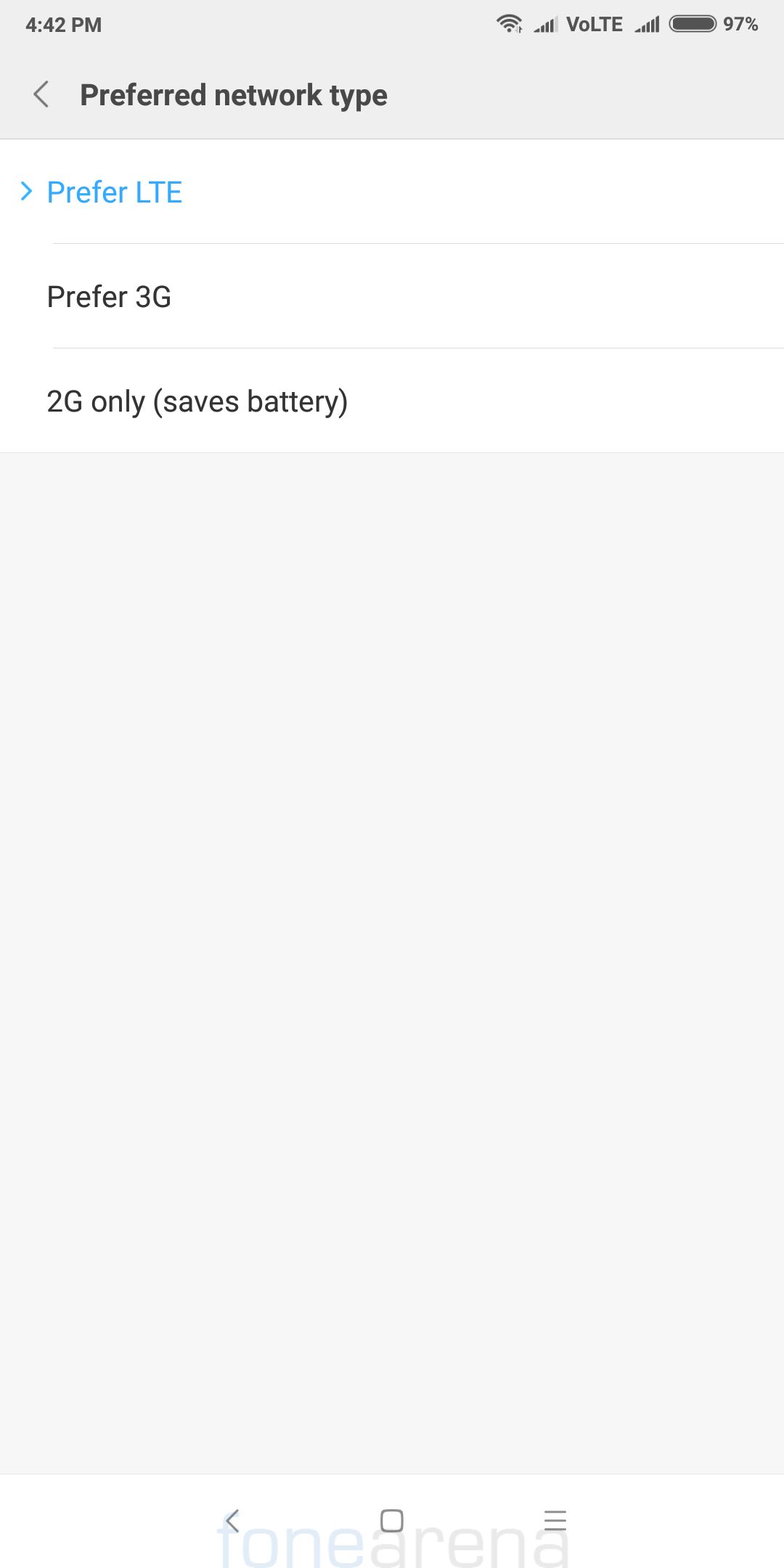This is a detailed screenshot of a mobile device's settings interface, taken at 4:42 p.m., as indicated by the timestamp at the top of the screen. The top bar also displays the Wi-Fi signal, battery icon, and a nearly full battery at 97%. Below the top bar, a black arrow icon pointing left is labeled "Preferred network type." Accompanying this text, a blue arrow pointing right leads to a highlighted option that reads "Prefer LTE" in blue letters, surrounded by other network options in black text. The alternatives include "Prefer 3G" and "2G only (saves battery)." There is a lengthy gray section with no content, leading to the Android navigation bar at the bottom of the screen, featuring a left-pointing arrow, a square, and a set of three short horizontal lines arranged in a square formation. The bottom of the screenshot bears a watermark that reads "FONEARENA." The image is devoid of any people, animals, plants, buildings, bridges, vehicles, or airplanes, containing only textual and graphical elements related to the phone's interface.